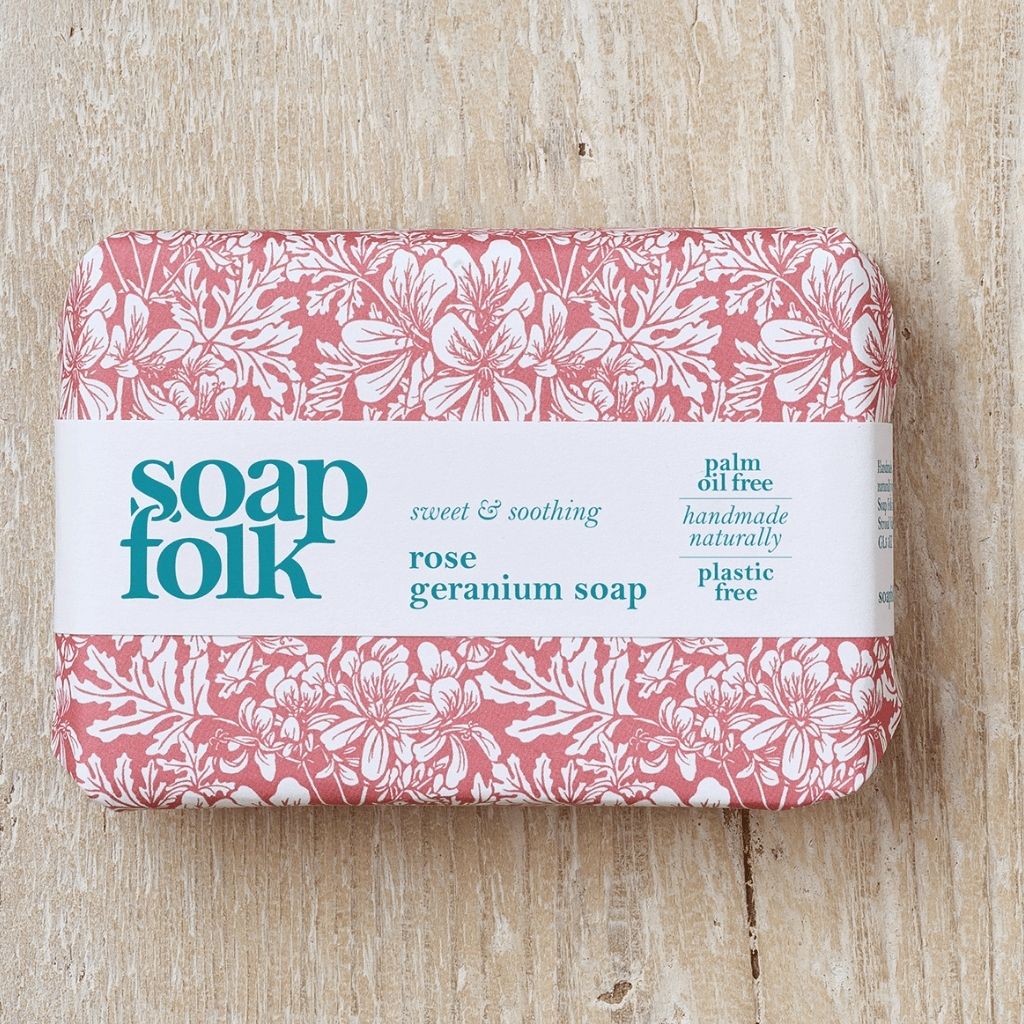This is a photograph of a beautifully wrapped bar of soap resting on a light beige, wood-textured surface with distinctive grain and almost white markings. The soap is encased in a decorative paper wrap, adorned with a delicate pattern of white flowers and oak leaves against a reddish-pink background, reminiscent of old woodcut prints. A white paper band encircles the soap at its center, displaying elegant teal lettering. The text reads:

- "Soap Folk" in large, prominent letters on the left,
- "Sweet and Soothing" in italic script next to it,
- "Rose Geranium Soap" below that in a standard font,
- And on the right side, vertically arranged text: "Palm Oil Free," "Handmade Naturally," and "Plastic Free."

The overall presentation is charming and feminine, with the vibrant floral design and the stylish typography enhancing its visual appeal. The photo's composition, captured from an overhead perspective, further accentuates the soap's meticulously crafted packaging and the rustic yet refined tabletop.